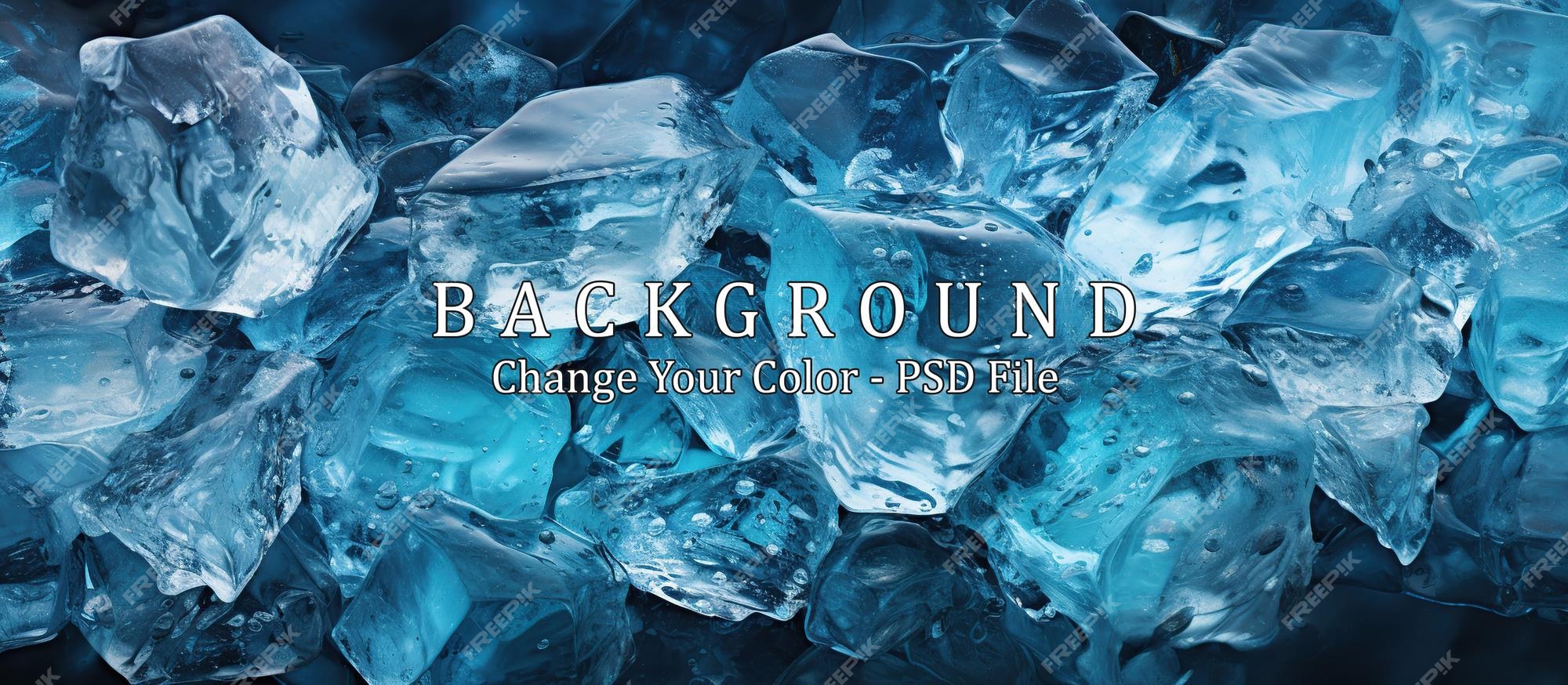This image appears to be promotional or an interface page, likely for a design-related product or resource. At its center, prominent white text reads "BACKGROUND" in bold, uppercase letters, with a smaller, lowercase subtext underneath that states, "change your color - PSD file." This text is superimposed on a backdrop that features an eye-catching composition of irregularly shaped ice pieces or translucent glass shards, primarily in shades of blue from light aqua to a deeper blue. These fragments are uneven, resembling anything from tiny chips to larger chunks and almost look as if they have been dynamically spewed from a ground formation. The jagged yet smooth pieces create an animated and vivacious aesthetic, further accentuated by the gradient from lighter to darker blues, particularly around the edges. The overall effect is vivid, almost as though the ice is alive and moving towards the viewer, making the image both visually stimulating and modern.